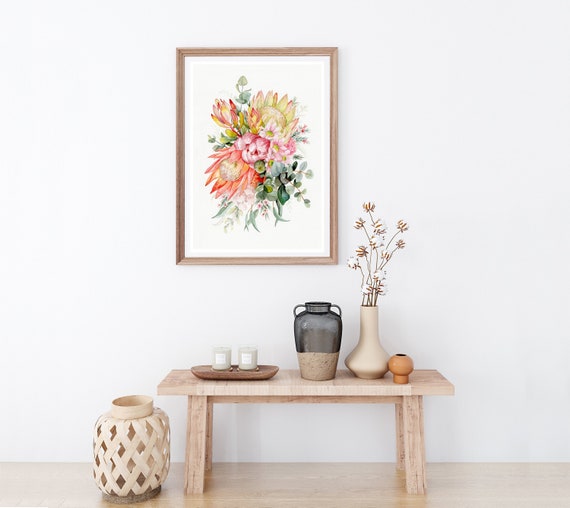This photograph showcases a meticulously staged interior of a house, emphasizing a minimalist yet elegant aesthetic. The backdrop features a pristine white wall adorned with a wooden-framed picture, vividly illustrating a colorful bouquet of flowers against a white background. Beneath this framed artwork sits a rustic wooden table that resembles a bench. Atop the table is an assortment of artfully arranged items: a vase filled with white, cotton ball-like plants, an urn-like vessel presumably for water, and a small tray holding two pristine white candles. To the left of the table, there is a decorative pot distinguished by a unique weaving pattern that incorporates perforations. The entire scene exudes a tranquil simplicity, designed to highlight an understated yet refined decor.